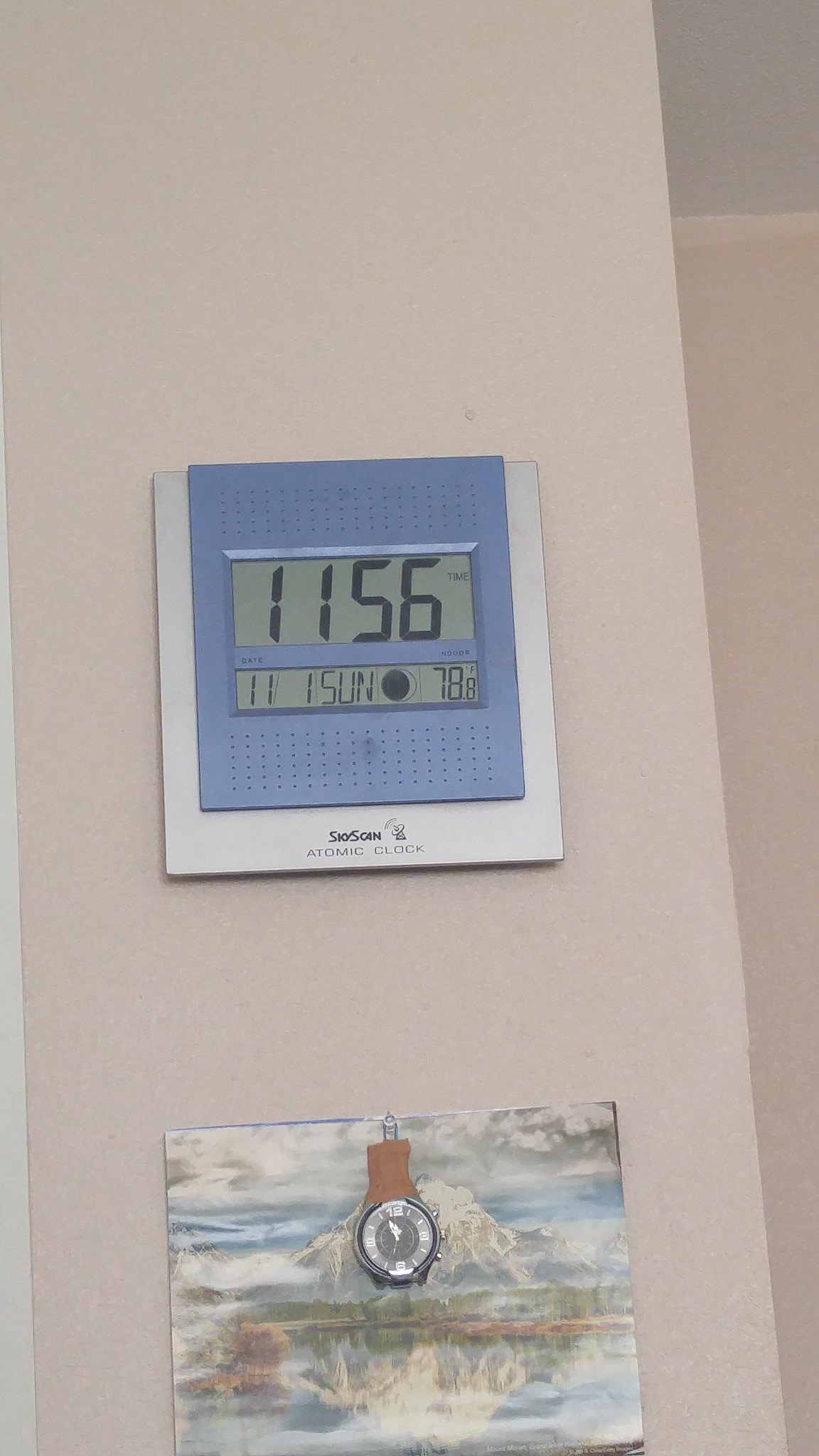In this photograph, which is vertically oriented, we see a cream-colored wall adorned with a few notable items. Prominently featured is a square, silver SIG scan atomic clock. The clock includes a blue faceplate with digital readings displayed in black text, indicating a temperature of 78.8 degrees, the word "Sunday," and the date "11." The time displayed on the atomic clock is 11:56. Below the clock hangs a muted-tone painting depicting a snowy mountain landscape. Draped over the painting is a wristwatch with a silver, round face, showing the time as approximately 11:35. The watch is attached by what appears to be a partial brown leather strap.